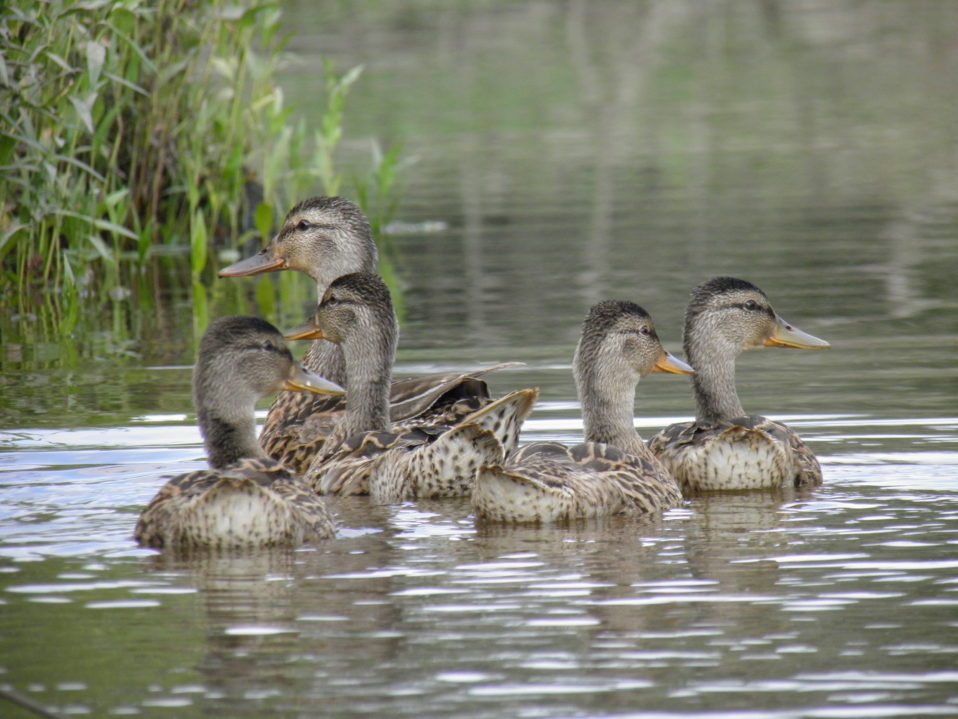In this outdoor image, a close-up captures five ducks swimming closely together on a sunlit body of water that might be a lake or river. The scene is detailed and vibrant, with the ducks' gray and brown speckled feathers standing out. The ducks exhibit varied behaviors: three look to the right and two to the left, their yellow-tinged beaks and speckled underparts adding to their distinct appearance.

The water around them ripples from their recent movement, with heavy reflections of sunlight glistening on the surface. In the background, reflective patches hint at trees, adding depth to the composition. Lush green reeds or weeds emerge from the upper left side of the image, their presence contrasting with the out-of-focus, stick-like reflections on the upper right.

One larger duck, possibly the mother, appears to be leading the group of four slightly smaller ducks, suggesting a familial arrangement. The viewing perspective is level with the ducks, ensuring they dominate the frame while the edges of the water remain unseen. This serene scene, bathed in daylight, illustrates a tranquil moment in nature.